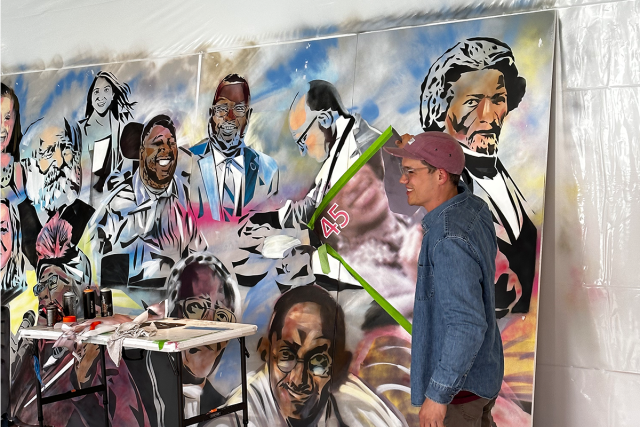In this detailed image, a young painter is captured in the midst of creating a mural, which prominently features historical figures, many of whom are Black. The painter, who is partly facing the camera with a smile, is dressed in a light red baseball cap, a denim jacket, khaki pants, and glasses. He is holding up a green-edged section of the mural, which intriguingly includes a man's chin. The mural itself is rich with figures in various attire, some in suits, historical garments, and robes, set against a dynamic background of swirling blue, brown, yellow, red, and white hues. The number "45" is clearly visible, slanting in red with a white outline, adding a striking element to the piece. In front of the mural, a white portable metal table with black ends is laden with artistic supplies, including an array of spray paint cans, rags, and stencils. This table sits against a wall protected by clear plastic sheeting, hinting at the meticulous care taken to preserve the surroundings from paint splatters. The mural's evocative style appears to connect various elements of Black history with a mix of figures, primarily dark-skinned, wearing white and blue clothing, illustrating a diverse and dynamic historical narrative.